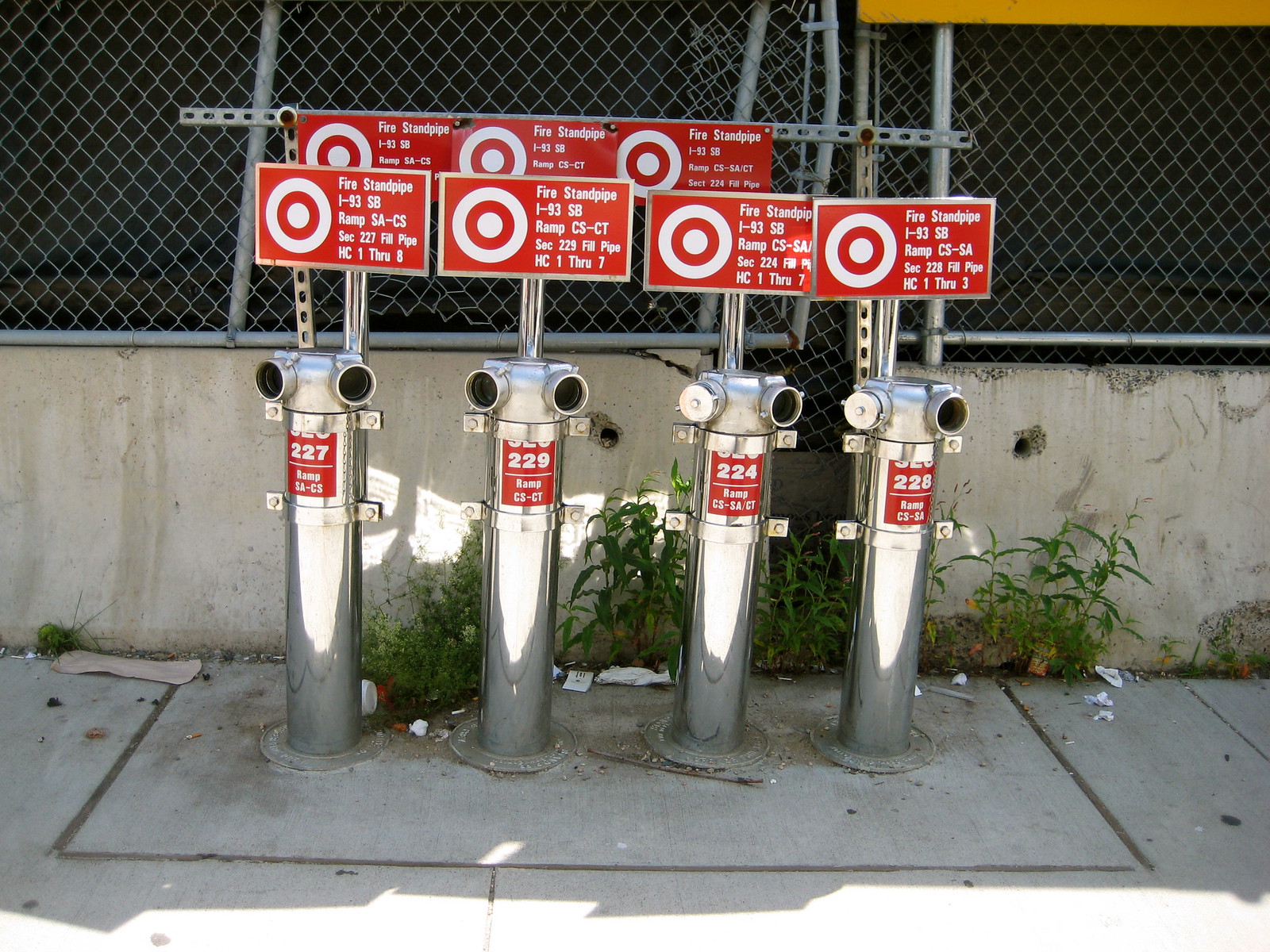The image depicts an outdoor scene featuring a sidewalk bordered by a waist-high concrete wall topped with a chain-link fence. Growing through the cracks in the pavement are several green weeds. At the forefront, four metallic fire standpipes, likely made of chrome or aluminum, extend vertically from the concrete ground. Each standpipe features two receptacles at the top, meant for connecting fire hoses. Above each pipe, there is a prominent red sign with a white target logo and the text "FIRE STANDPIPE." The signs also display various identifiers, including numbers such as 224, 227, 228, and 229, and detailed location information such as "I-93 SB ramp CSCT" and "Section 228 Field Pipe HC1 through 3." The overall scene is both industrial and functional, highlighting the preparedness for emergency fire-fighting operations.